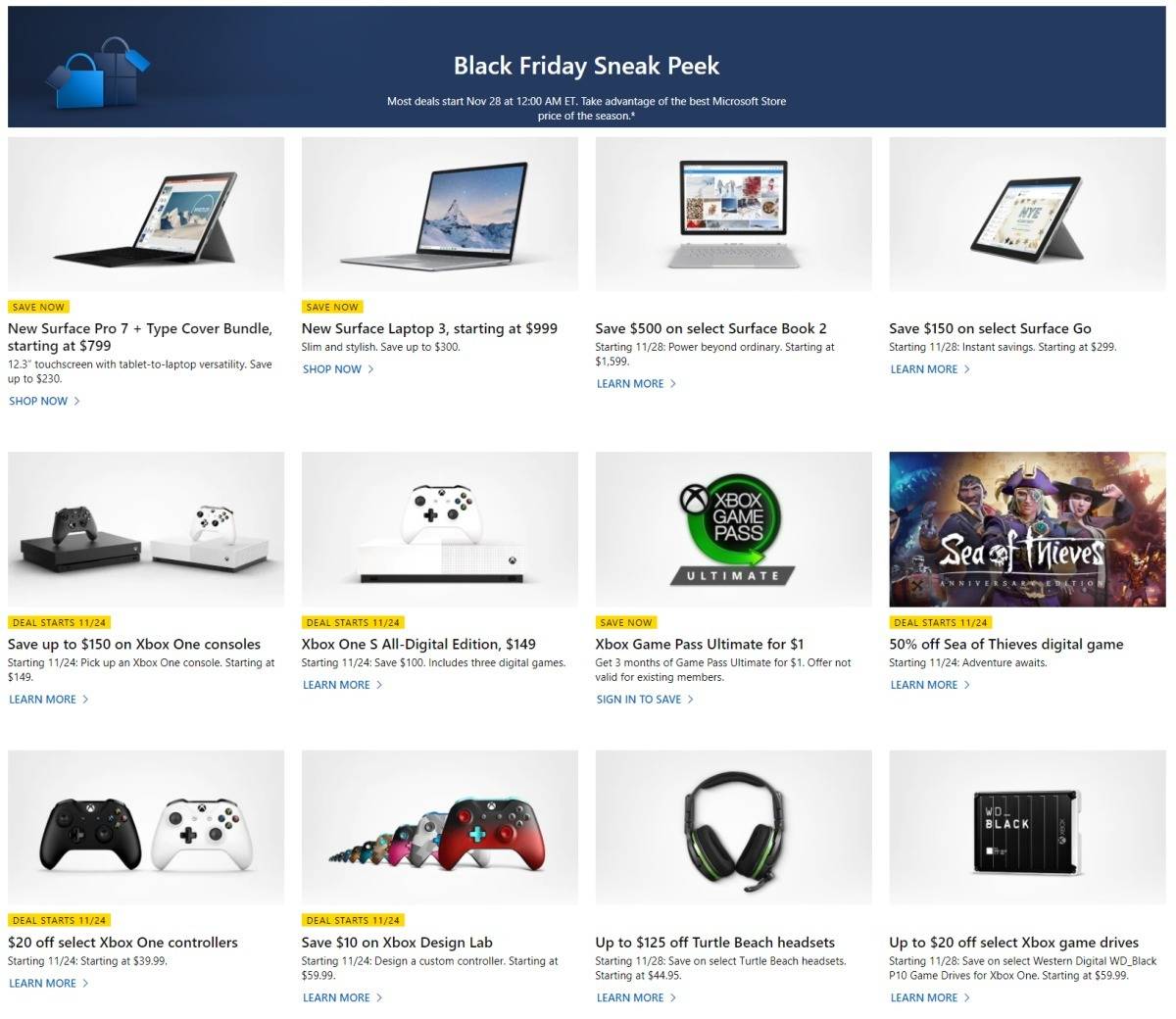This is a detailed caption of the provided web page image:

The top section of the web page features a blue strip with the title "Black Friday Sneak Peek" prominently displayed in white text. In the top left corner, there are two blue shopping bags. Below the main title, a subtext reads, "Most deals start November 28th at 12am ET. Take advantage of the best Microsoft Store prices of the season."

The main body of the page is organized into four columns and three rows, displaying a variety of products. These include laptop computers and Surface Book tablets, computer games such as "Sea of Thieves," an Xbox Game Pass, Xbox consoles including the Xbox One S and Digital Edition, various game controllers, Xbox One controllers, Turtle Beach headsets, and Xbox Game Drives. Yellow labels are attached to many of these items, indicating promotions with text such as "Save Now" or specifying the date deals begin, like "Deal Starts 11/24."